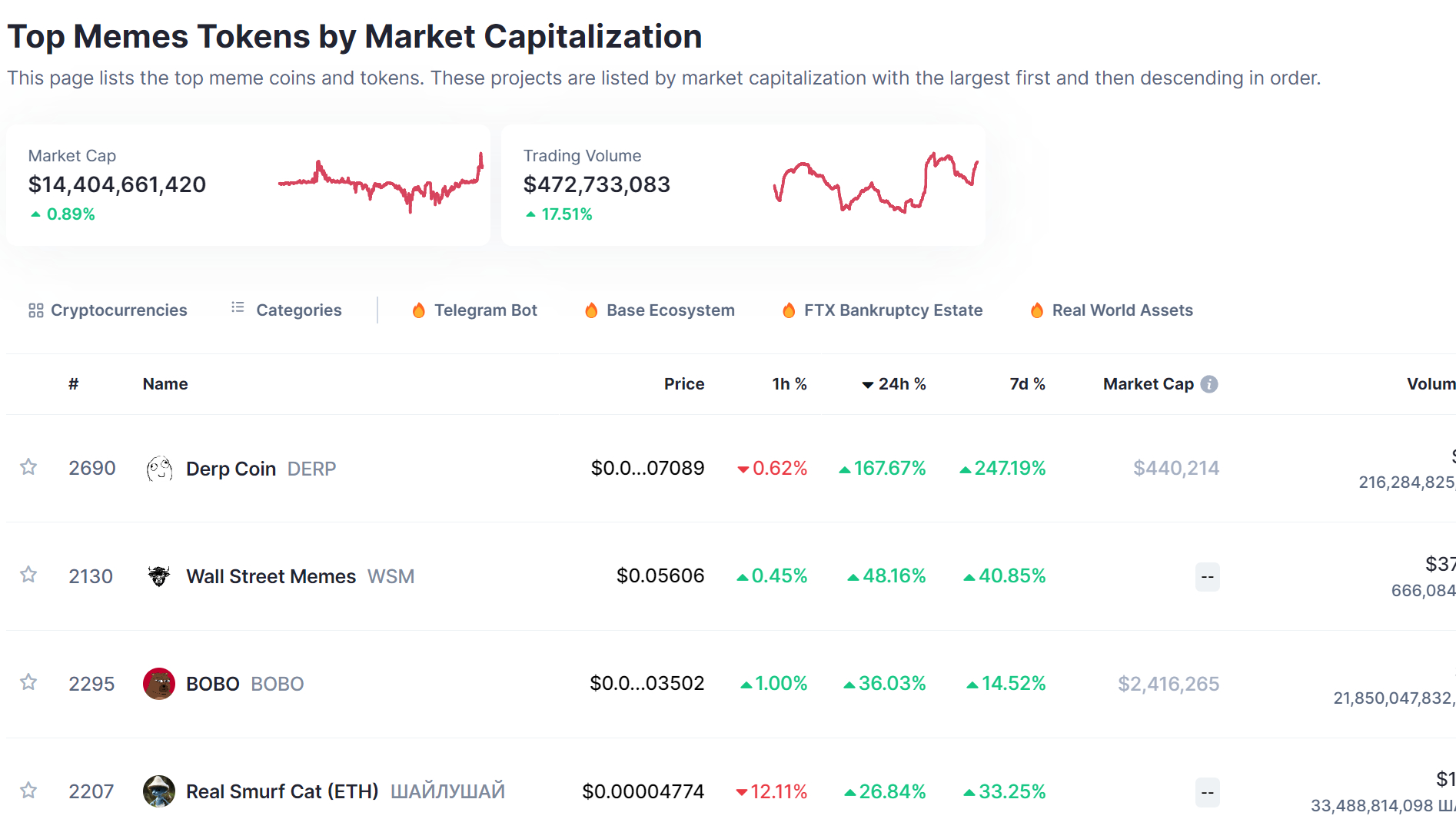**Caption:**

The webpage showcases a detailed spreadsheet listing the top meme coins and tokens ranked by market capitalization. At the top, it displays essential market statistics: the total market capitalization stands at $14,404,661,420, which has seen an increase of 0.89%. Additionally, the trading volume is $472,733,083, up by 17.51%. The page features a tracking chart with ticker lines indicating market movements, highlighting recent trends with red zigzag lines showcasing fluctuations.

The site categorizes cryptocurrencies into various segments such as "Telegram Bot", "Base Ecosystem", "FTX Bankruptcy Estate", and "Real World Assets." Below this section, there's a detailed spreadsheet with columns labeled "#", "Name", "Price", "1h %", "24h %", "7d %", "Market Cap", and "Volume". Some of the meme coins listed include Derpcoin, Wall Street Memes, Bobo, and Real Smurf Cat ATH.

The data reveals significant volatility: Derpcoin experienced a slight decline of 0.62% over the past hour but saw a tremendous increase of 167% in the past 24 hours. Meanwhile, Wall Street Memes surged by 48% in the same timeframe. Real Smurf Cat ATH displays a dramatic drop of 12.11% in the past hour, although it’s up nearly 27% over the past day. The figures illustrate the wild fluctuations and unpredictable nature of these meme tokens, emphasizing the unpredictable and often chaotic nature of the meme coin market.